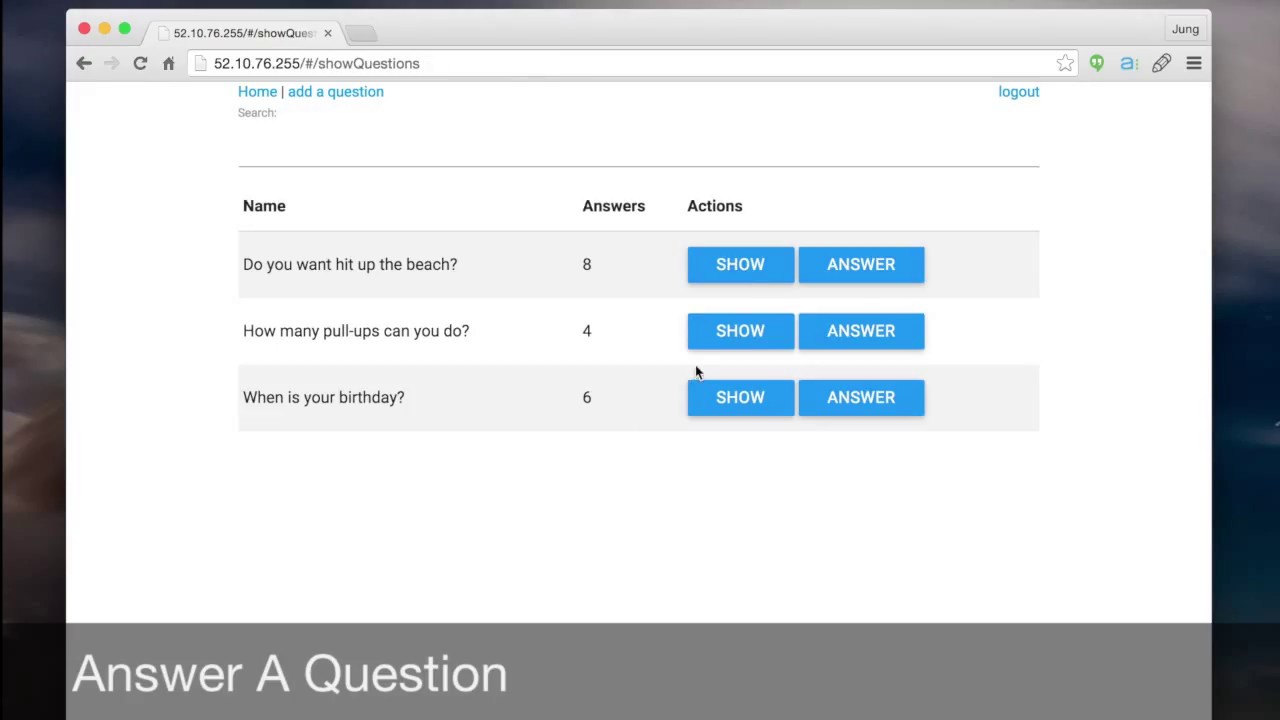Here is a cleaned-up and more detailed description:

---

A screenshot of a partially visible website is displayed against a faintly cloudy, blue-tinted background, which occupies the edges of the image. The site doesn’t fill the entire screen, creating a border effect reminiscent of a serene sky.

In the top-left corner of the browser's window, there are the typical red, yellow, and green dots indicating window controls, accompanied by a tab labeled "52.10.76.255/#bashflashshowquestions". Opposite this, on the top-right, the text "Jung" is visible, possibly indicating the user’s name or a feature of the site.

Directly beneath this, the browser toolbar includes common navigation icons: a back arrow, a forward arrow, a refresh button, and a home icon. The address bar repeats the URL "52.10.76.255/#bashflashshowquestions", and to its right are a favorites button, an edit button, and an options button represented by a three-line icon (often referred to as a hamburger menu).

The main interface of the website presents several interactive elements: a menu bar displaying "Home," "Add Question," and "Log Out" in blue text, followed by a search bar. Below this, the content is organized into three columns: "Name," "Answers," and "Actions."

- Under "Name," the entries are "Do you want to hit up the beach?", "How many pull-ups can you do?", and "When is your birthday?"
- Corresponding to these names, the "Answers" column shows "8," "4," and "6" respectively.
- The "Actions" column includes identical buttons labeled "Show Answer" for each entry.

A gray border frames the bottom of the content area, providing a clean separation from the rest of the webpage.

---

This detailed caption provides an accurate and comprehensive description of the website screenshot, including layout, elements, and content.